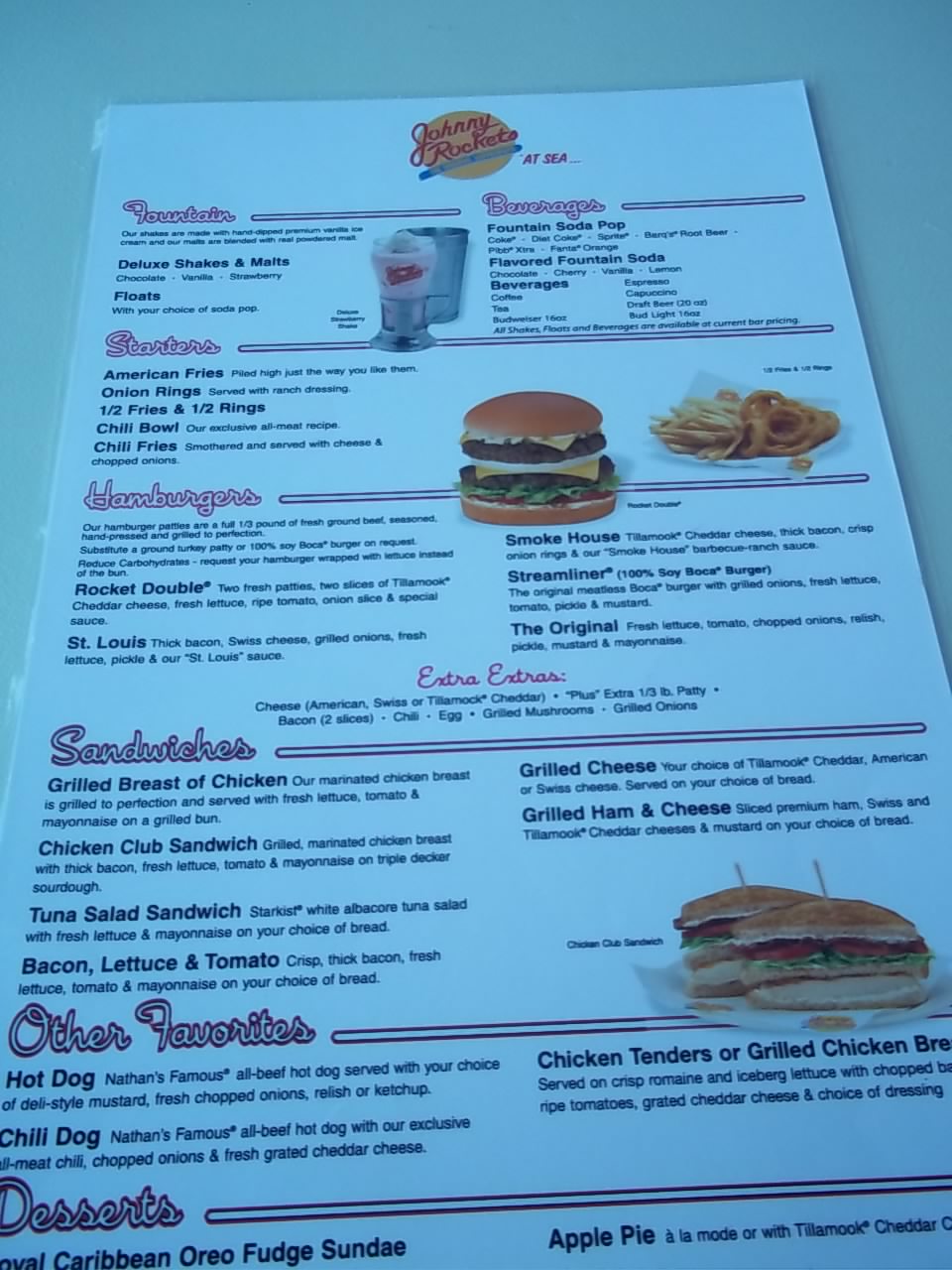This detailed image captures the full front page of the Johnny Rockets menu, prominently displayed on what appears to be a white piece of paper laid on a table. The menu is quite extensive, packed with a wide array of delectable offerings. 

At the very top, the menu lists an assortment of beverages including deluxe shakes and malts, floats, fountain soda pop, and flavored fountain sodas. This is followed by the starter menu, featuring classic American appetizers like American fries, onion rings, chili bowl, and chili fries.

Next on the menu are the hamburger selections showcasing items such as the Rocket Double, St. Louis Smokehouse, Streamliner, and the iconic Original burger. The sandwich section comes next, offering options like a grilled breast of chicken sandwich, chicken club sandwich, grilled chicken, and a grilled ham and cheese sandwich.

Following that, the menu highlights other favorite items such as hot dogs, chili dogs, and chicken tenders. Finally, it rounds off with a variety of tempting desserts.

The menu is visually appealing with numerous images of their popular dishes including hamburgers, onion rings, sub sandwiches, and milkshakes, making the selection process even more enticing. This comprehensive menu truly showcases the expansive and delicious offerings of Johnny Rockets.